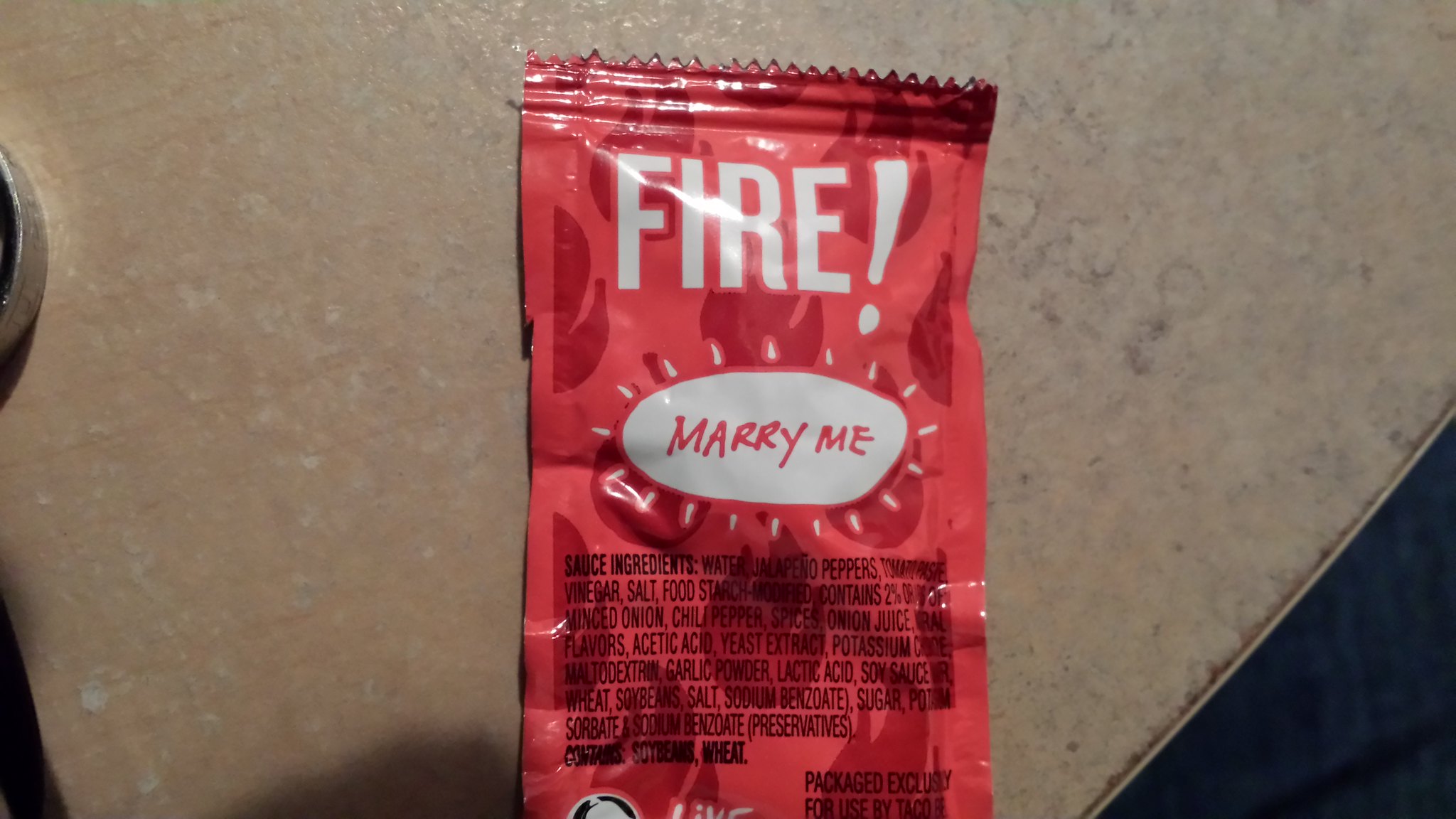The image depicts a red packet of sauce adorned with fire illustrations in various shades of red. The top of the packet features a zigzag pattern, indicating its opening mechanism, and prominently displays the word "FIRE!" in bold, white, all-uppercase letters. Below this, within an outlined white oval, the text "Marry Me" is printed in red. The lower section of the packet is densely packed with a detailed list of ingredients, which includes water, jalapeño peppers, tomato paste, vinegar, salt, food starch, onions, chili pepper, spices, onion juice, maltodextrin, flavors, acetic acid, yeast extract, potassium chloride, garlic powder, lactic acid, soy sauce (containing wheat, soybean, and salt), sodium benzoate, sugar, potassium sorbate, and additional preservatives. Notably, it mentions the inclusion of soybeans and wheat. At the bottom, there is a small white icon with the text "LIVE" printed inside it. The packet is placed on a light brown marble or granite surface, with a darker area in the bottom right corner and light reflecting off the top of the packet.